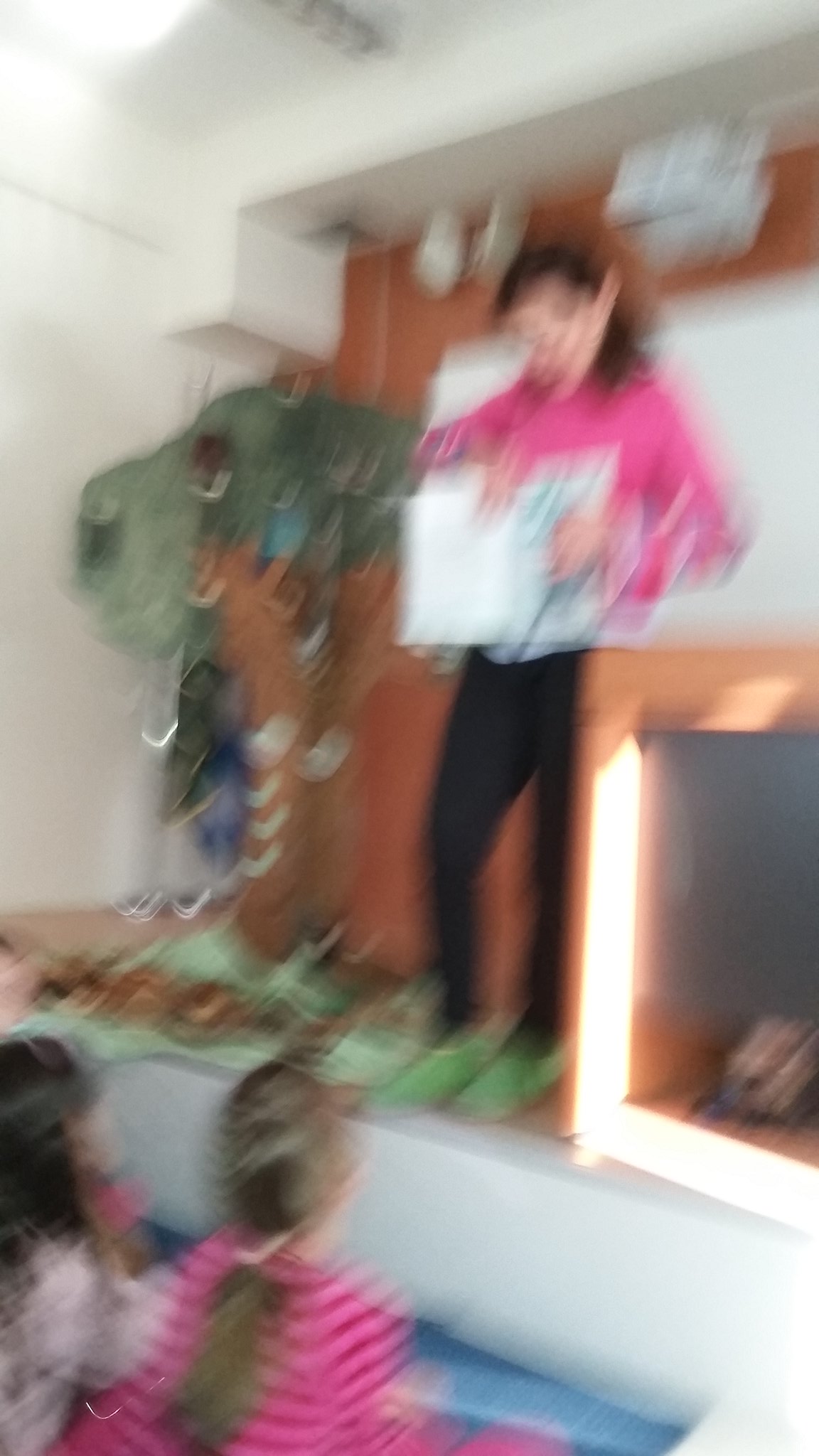In this blurry vertical image, a female teacher stands on a platform, surrounded by a group of attentive children aged around eight or nine. All participants are Caucasian. The teacher, clad in dark pants, green athletic shoes, and a magenta pink sweater, gazes down as she holds a box. Flanking her are a tree prop and what appears to be a large, thick box or a mock fireplace, adding to the scene's theatrical atmosphere. Above her, a cutout in the wall, enhanced by built-in stage lights and a speaker, gives the area a stage-like appearance. Among the children, a girl with long blonde hair tied back in a ponytail wears a dark and light pink horizontally striped shirt. Another girl with dark hair and a headband sports a light-colored, long-sleeved shirt. The floor in front of the children is blue.